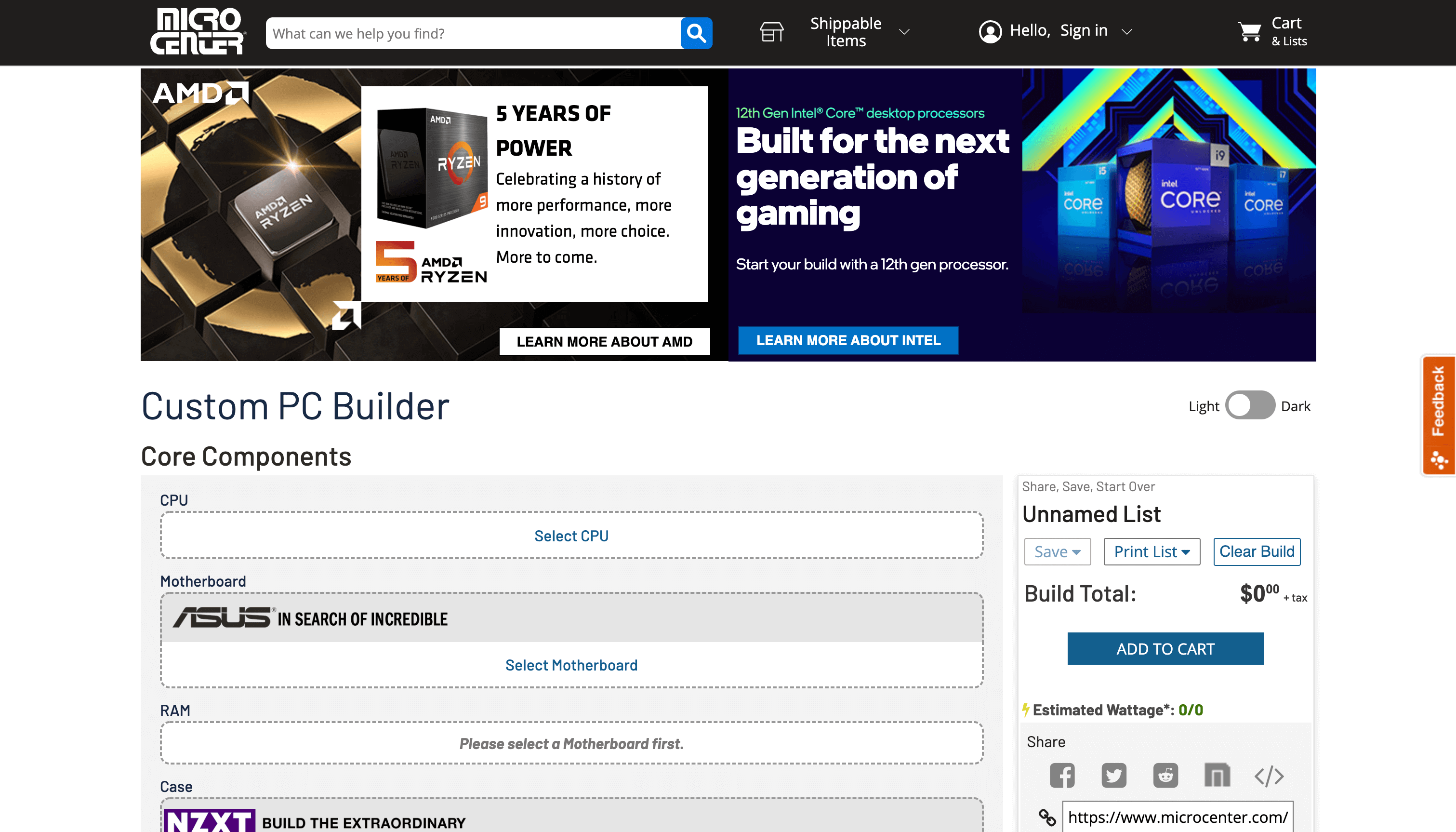The screenshot depicts a webpage from the Micro Center website, known for its comprehensive selection of computer components and electronics. In the top left corner, the stylized Micro Center logo is prominently displayed. To its right, a search bar invites users to explore the site with the prompt, "What can we help you find?" Adjacent to the search bar, tabs for "Shippable Items" and "Hello, Sign In" are visible, followed by an icon representing the user's cart and any user-created lists.

Beneath this navigation bar is a prominent banner advertisement highlighting Horizon products, emphasizing "five years of power" and celebrating a history of "more performance, more innovation, more choice, more to come." Next to this is another advertisement promoting the 12th Gen Intel Core desktop processor.

Further down, the site features a "Custom PC Builder" section, offering a personalized computer assembly option. Users can switch between light mode and dark mode for the website, and an unnamed list is visible. The left side of the screen provides options for selecting various PC components. The CPU and motherboard fields indicate that nothing has been selected, with a notable advertisement for Asus motherboards. Clarification is provided below these fields, stating that the motherboard must be chosen first before selecting RAM. The case selection option appears, but is partially obscured by an advertisement for NZXT cases.

Overall, the Micro Center website provides users the ability to not only purchase individual computer parts but also offers tools and advertisements to assist in custom building their own PCs, likely catering to both hobbyists and professionals seeking high-performance hardware solutions.